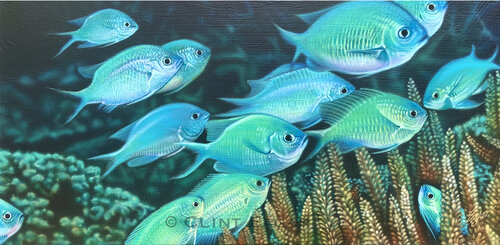This detailed underwater panorama photograph captures approximately 10 to 12 tropical marine fish amid a vibrant aquatic landscape. The elongated image is about twice as wide as it is tall, emphasizing the depth and range of the underwater scene. The fish, characterized by their tall, narrow bodies with a silvery blue-green metallic sheen, swim predominantly towards the right side of the image. Their small, round, black eyes, together with their forked Y-shaped tails and small dorsal fins, are finely detailed. Notably, two fish on the right side of the photo face left, slightly trailing the others.

In the lower right corner, golden-yellow and orange underwater plant life with long, thin fronds and smaller offshoots stand out, adding a splash of contrasting color. The blurred rear background reveals a mix of blue and dark teal hues, dotted with out-of-focus anemones and branched corals on the left side. The presence of these reefs and corals provides a textured backdrop to the primary subject, the school of fish, immersed in this serene marine habitat. The entire scene is artistically composed, evoking a sense of tranquility and natural beauty, as though the viewer is witnessing a snapshot of life beneath the waves.